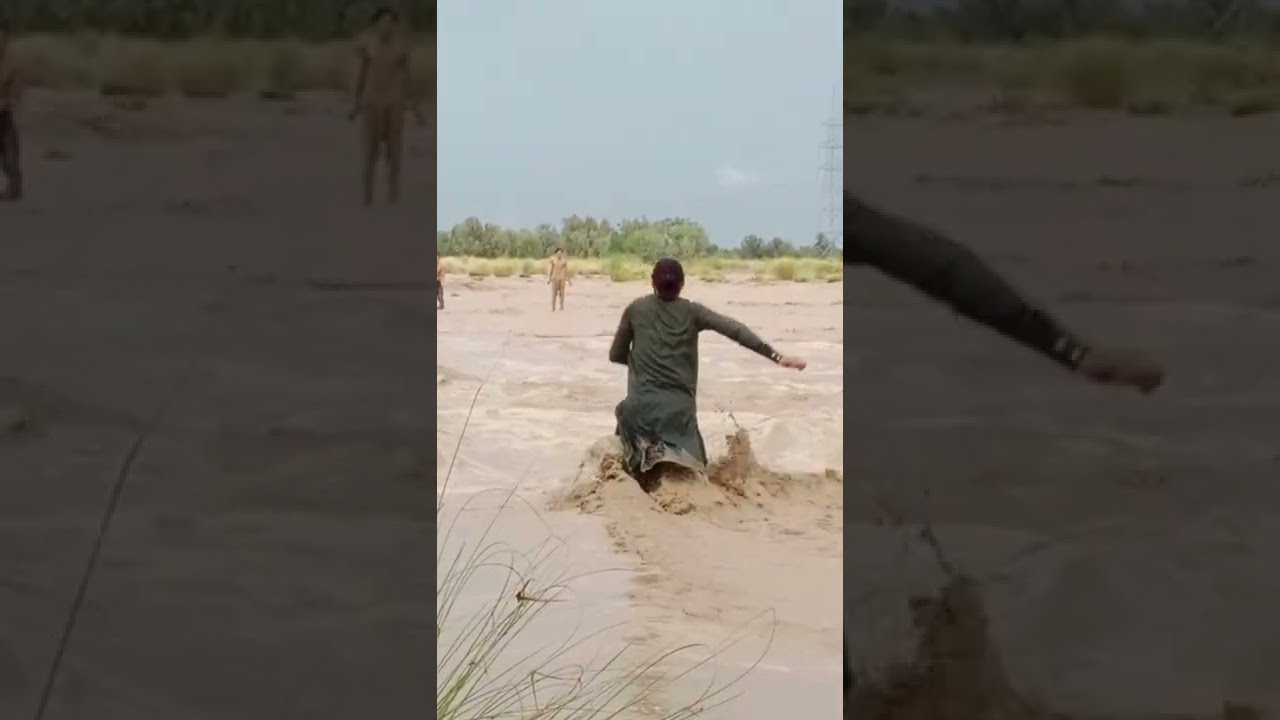In this striking image, a woman with dark hair, dressed in a very dark green or possibly brown outfit, is struggling to navigate through knee-high, turbulent, muddy water that splashes around her. The scene captures her mid-motion as she heads towards a sandy shoreline, her arms swinging as though she is struggling with the difficult crossing. In the background, a man can be seen standing shirtless on the shore, watching her. Further back, a lush green tree line extends across the image, with a bright blue sky peeking through behind the greenery. The main photo is presented vertically down the middle of the composition, while the left and right sides feature zoomed-in, grayscale versions of the same image. On the left side, there’s a closer view of the standing man and some long green grass, while the right side focuses on the woman’s arm and the turbulent water swirling around her.